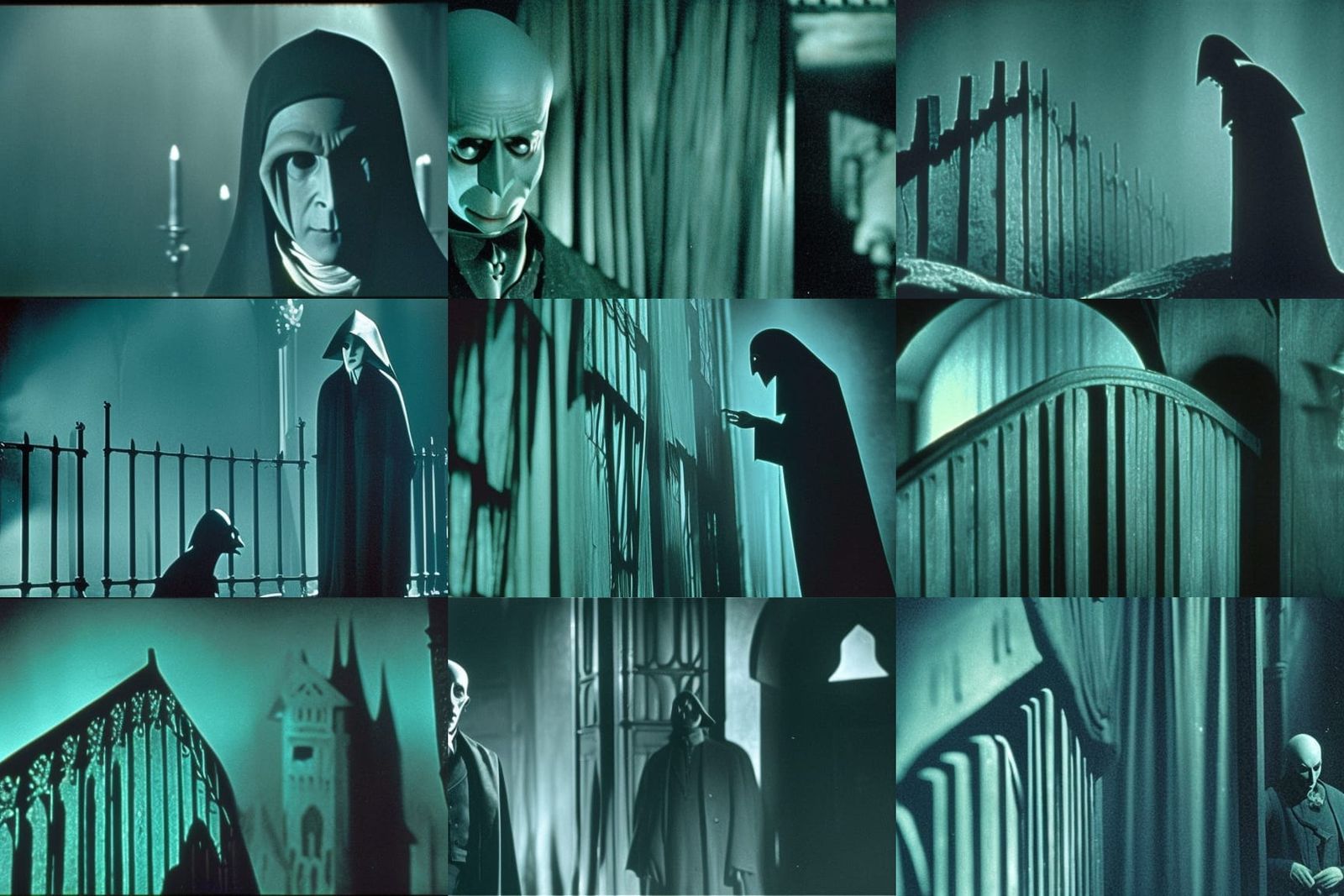Here’s a detailed descriptive caption for the series of images:

---

This rectangular montage, formatted in a landscape orientation, appears to be a collection of frames from an animated claymation film, possibly a movie or a video game cutscene. The sequence, comprising nine images, features a dark, mysterious, and somewhat eerie aesthetic dominated by shades of blue and black, with a hazy atmosphere.

1. **Top Left:** The first image depicts a nun-like figure with a fixed habit covering her head, her face altered to resemble an alien with large, protruding eyebrows and a sharp nose. Flickering candles illuminate the background.

2. **Top Center:** In the second frame, a man with a steampunk or vintage suit and tie is shown with his chin dipped down. He is bald and has an otherworldly appearance, featuring exaggerated sharp features. The backdrop consists of heavy curtains.

3. **Top Right:** The third image portrays a figure in a Paul Revere-style hat and cloak, slightly leaning forward and gazing down at a fence. A thick fog further shrouds this dimly-lit scene, enhancing its mysterious aura.

4. **Middle Right:** This frame zooms in on a textured fence, allowing viewers to appreciate the intricate details and the overall dark and foggy ambiance of the series.

5. **Bottom Right:** A man in a suit stands in the bottom corner, while the camera focuses on a textured surface, possibly curtains or paneling. The depth of field highlights the man’s subdued presence in this enigmatic environment.

6. **Bottom Center:** In this frame, at least two characters are visible. A bald man in a suit, likely recurring throughout the series, stands alongside a figure in a black mask. The setting suggests an indoor location or just outside a building.

7. **Bottom Left:** This image is an unclear depiction of what may be a distant tower or a close-up of a fence. A potential hooded figure adds an element of intrigue to the scene.

8. **Middle Left:** The nun reappears in a full-body shot. She stands while a bald, kneeling figure at her feet, possibly the same man from the previous images, enhances the unsettling atmosphere.

9. **Center:** The final, central image focuses on a figure, potentially the nun, leaning forward. Clad entirely in black, with a white hand extending an index finger, the figure points towards what might be a building, encapsulating the creepy tone that permeates the entire series.

---

This collection captures a haunting, macabre narrative through a blend of surreal characters and dim, fog-laden settings, each frame contributing to the overall eerie and enigmatic atmosphere.